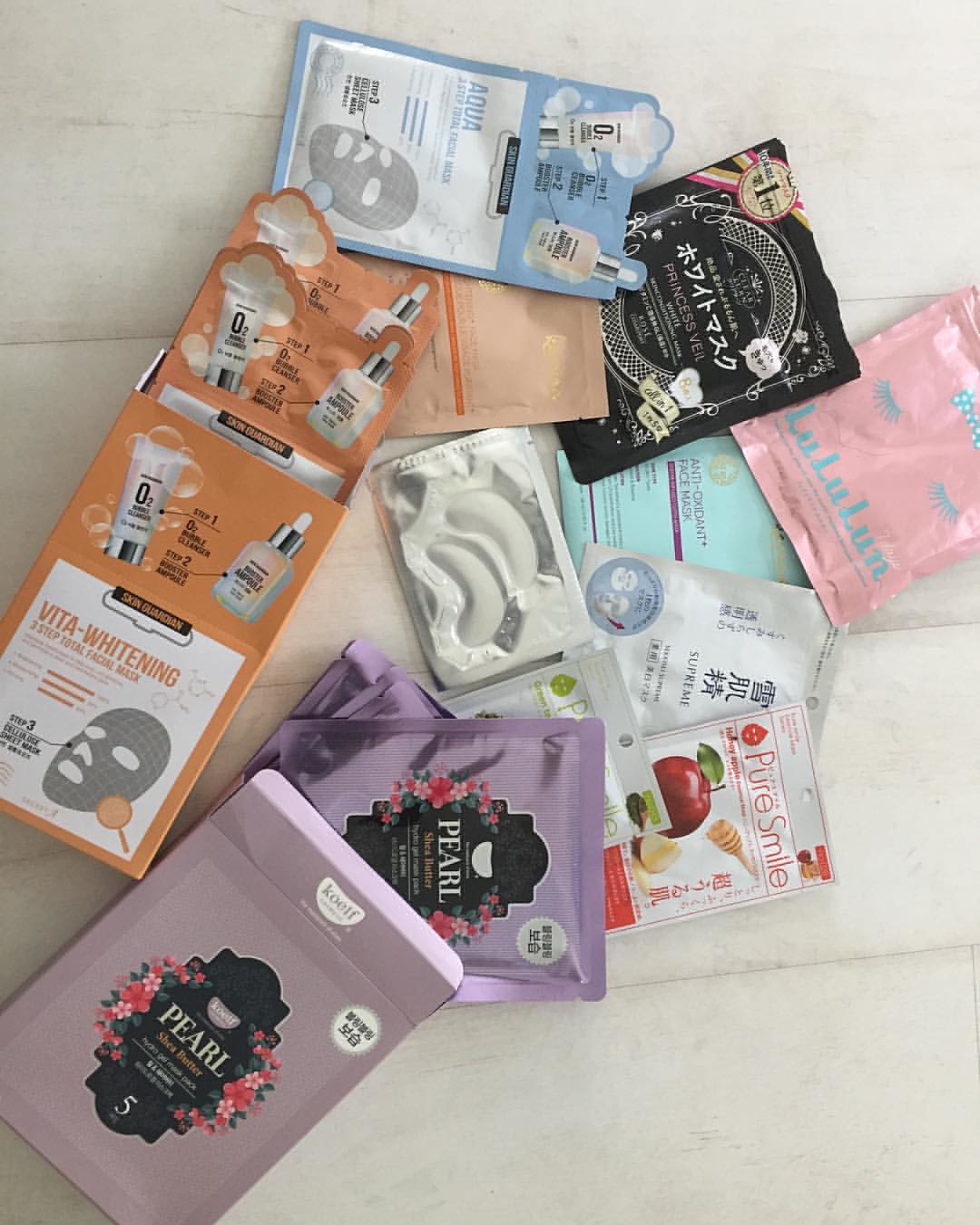This photograph features an array of cosmetic products meticulously laid out on a table, each in flat packaging. Centered in the display is an orange box labeled "Vita Whitening 3-Step Total Facial Mask," which includes an illustration of the mask and text primarily in English, with additional Asian characters. Adjacent to it is a purple package labeled "Pearl Shea Butter," also featuring small Asian script. Another standout in the collection is a sleek black package titled "Princess Veil White," adorned with Asian characters as well. The arrangement also includes an aqua-colored facial mask package, mirroring the design of the orange Vita Whitening box but in a blue hue. The cohesive display highlights an assortment of facial masks, characterized by a blend of English and Asian text, suggesting an international selection of beauty products.